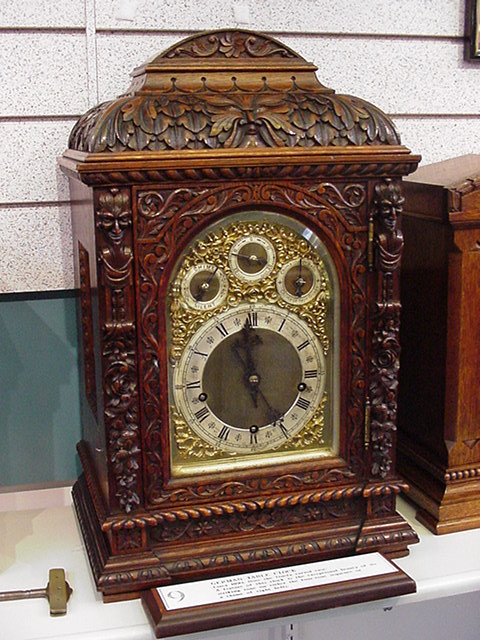This image features a beautifully crafted antique mantel clock, positioned on a pristine white countertop. The backdrop includes a bluish wall adorned with textured paneling, adding a touch of vintage charm to the scene. The clock itself is a rectangular masterpiece, meticulously carved from wood. Faces and figures intricately enhance its trim, showcasing remarkable artisan skill. 

The base of the clock tapers outward, providing a sturdy foundation, while the top narrows and culminates in a softly rounded pinnacle. The wood varies in hue, with the upper section displaying a light, woodish brown, and the lower front exuding a rich, deep brown. 

The clock face stands out with its unique shape, combining a rectangular form with a rounded apex. It features a gold background and a dark grey face, accentuated by a white circle that displays the numbering. Above the main face, three smaller dials mirror this elegant design, contributing to the clock's sophisticated appearance. 

To the right edge of the image, the corner of another wooden clock is faintly visible, hinting at a collection of timeless pieces.